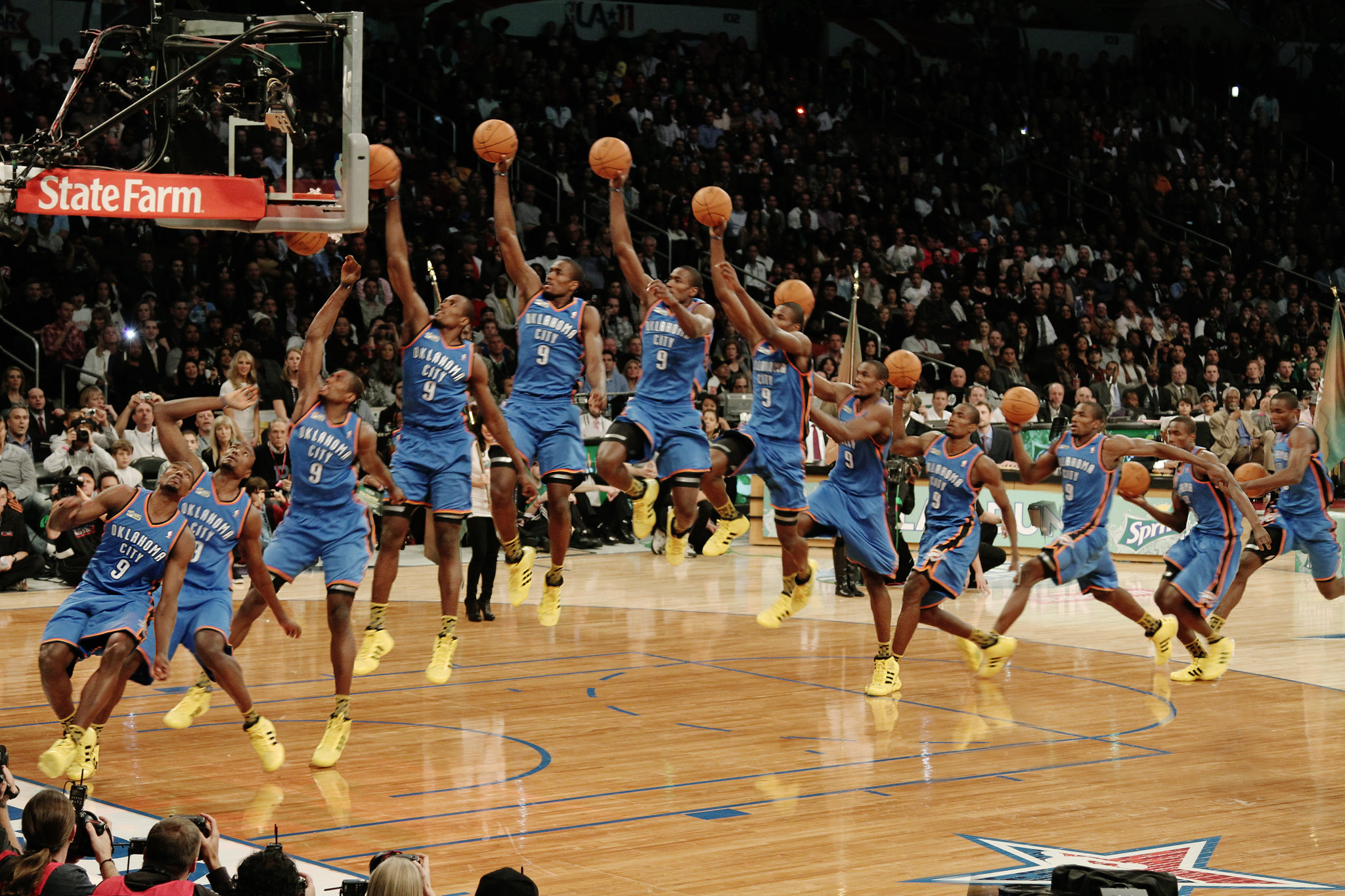In this composite photograph, an African-American basketball player, wearing a blue Oklahoma City jersey with the white number nine and yellow Nike high tops with black trim, is shown executing a dunk. The still image captures twelve sequential frames, stitched together to depict the player dribbling, running, leaping, and dunking the ball. In each frame, the athlete's position advances towards the hoop, illustrating his fluid motion towards the net. The scene is set in a sold-out arena, filled with spectators capturing the moment, highlighting the significance of the event. The basketball hoop features State Farm branding, adding a commercial touch to the energetic and dynamic composition.